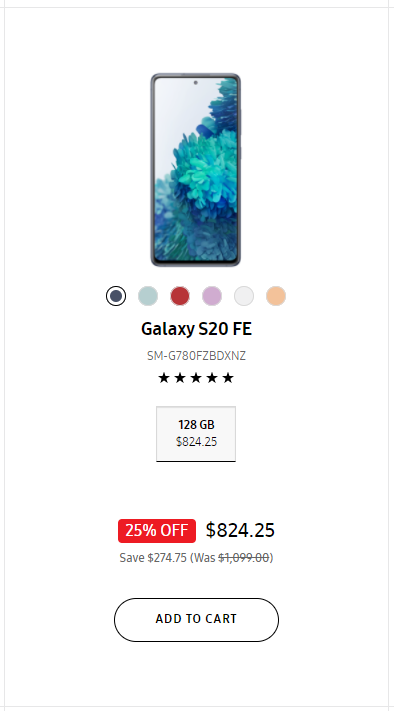The image appears to be a screenshot from a smartphone, likely displaying an online shopping page for a mobile device. The background is predominantly white, creating a clean and minimalistic look. At the top of the screen, there is an image of the phone in question, which showcases a close-up photo of green tree leaves against a backdrop of sky in the upper left corner.

Below the main image, there are several color options for the phone, including black, light blue, red, pink, white, and peach. Beneath these color choices, the product name "Galaxy S20 FE" is prominently displayed, alongside the model number "SM-G780FZBDXNZ." This section also features a five-star rating, indicating high customer satisfaction.

Further down, there is a box that specifies the storage capacity of the phone, which is 128GB, and the price of $824.25. The price information is followed by a red rectangular banner that says "25% off," drawing attention to the discount. To the right of this banner, the original price of the phone, $1,099, is crossed out, emphasizing the savings of $274.75.

At the bottom of the screenshot, there is an oval-shaped "Add to Cart" button, inviting users to proceed with their purchase. Overall, the image is a detailed view of a shopping page for the Galaxy S20 FE, highlighting its key features, color options, pricing, and discount offer.